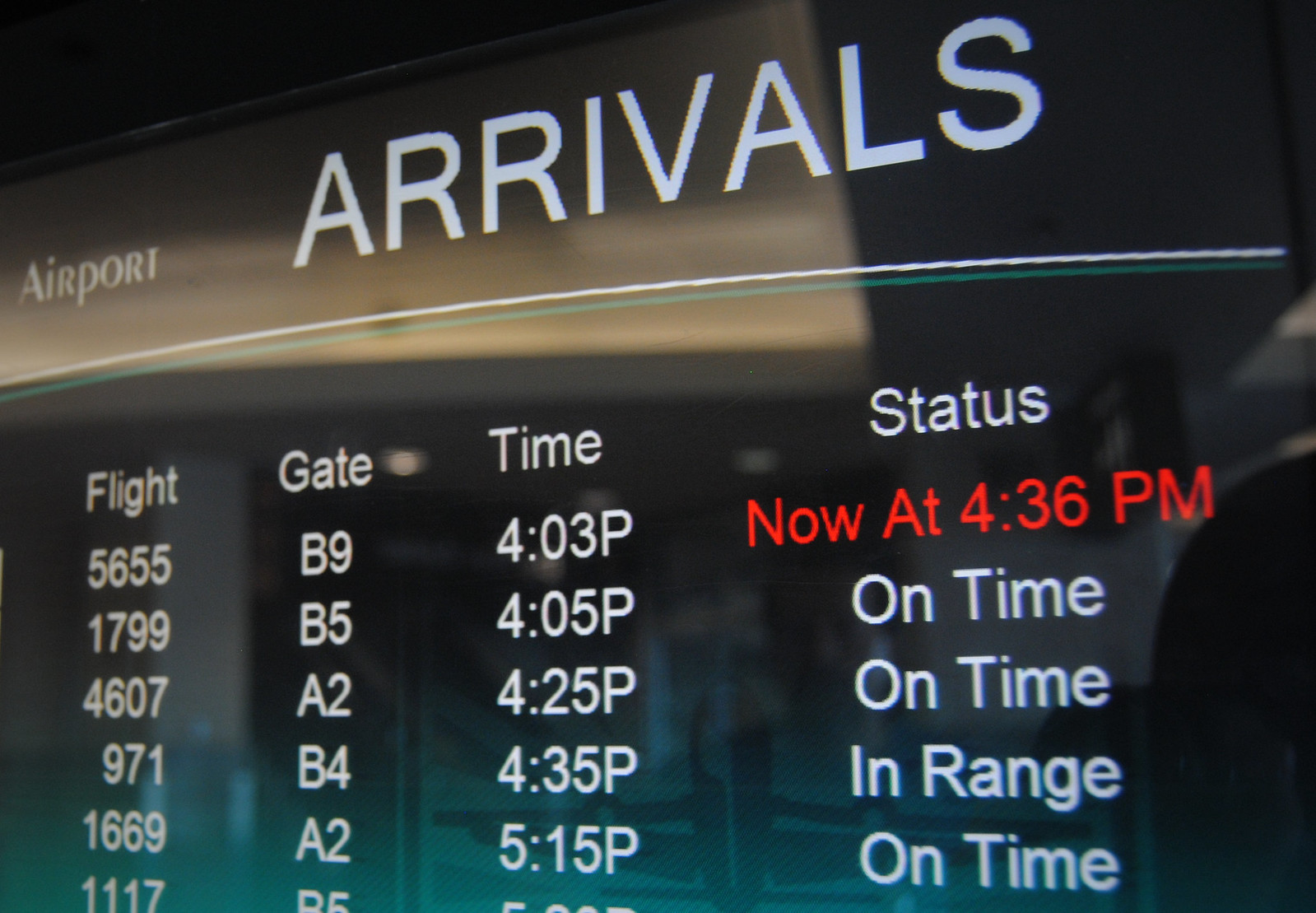This photograph shows the arrivals sign at an airport, featuring a dark background with a slight teal gradient. In the top left corner, the word "airport" is displayed in small white font. Adjacent to that, "ARRIVALS" is prominently shown in large all-caps white font. The sign details the flight number, gate, time, and status of arriving flights in neatly arranged columns.

The first flight listed is 5655 at gate B9, scheduled for 4:03 p.m., but its status is marked in red as "now at 4:36 p.m." The second flight, 1799, is arriving at gate B5 at 4:05 p.m. and is marked as "on time." Following that is flight 4607 at gate A2 at 4:25 p.m., also "on time." The fourth flight, 971, is set for gate B4 at 4:35 p.m. with the status "in range." Finally, flight 1669 is arriving at gate A2 at 5:15 p.m. with a status of "on time."

This comprehensive display provides travelers with crucial information about arriving flights, ensuring effective and timely communication.